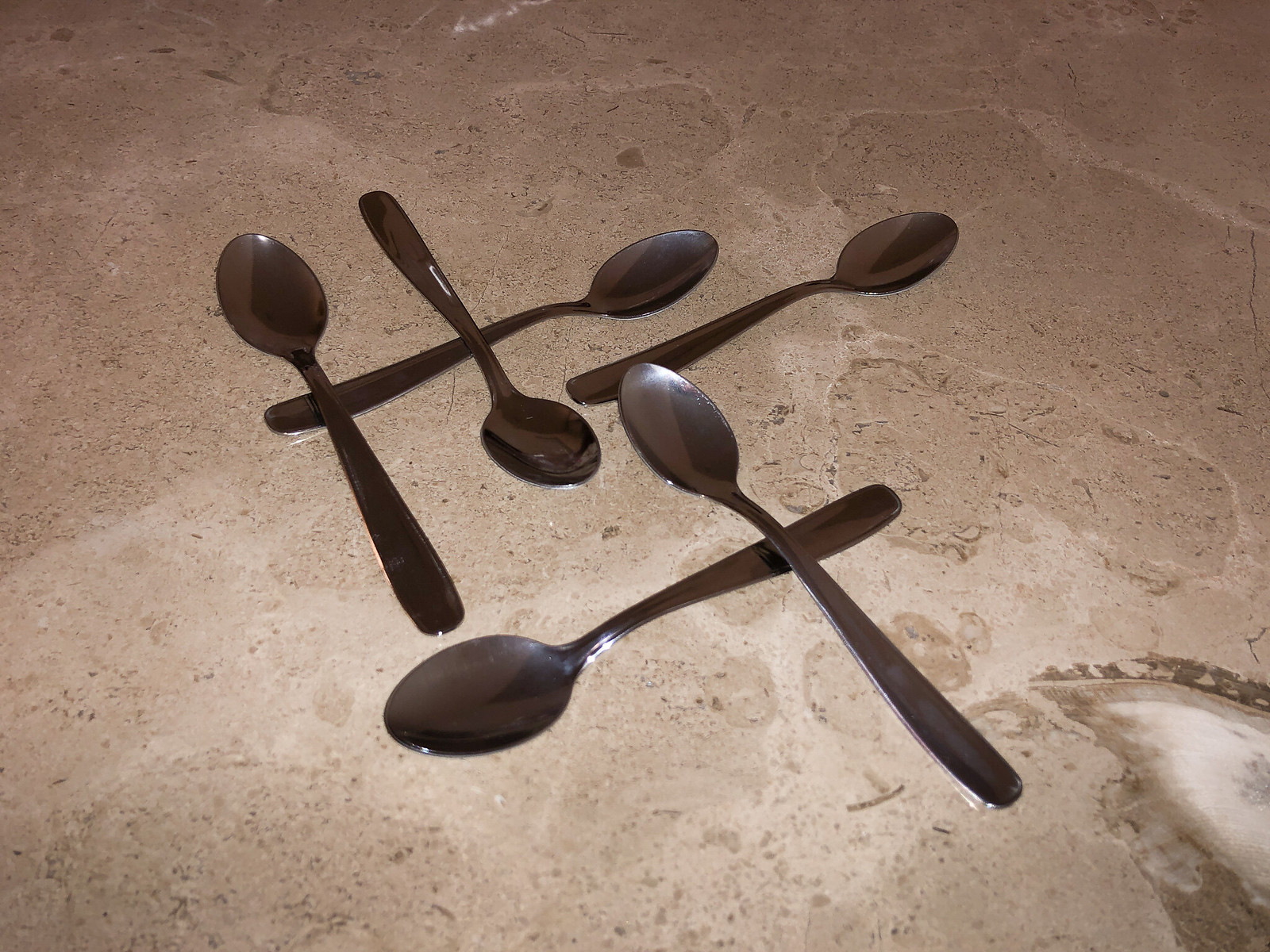The image is a color photograph featuring six silver teaspoons meticulously arranged on a flat surface that appears to be either travertine, marble, granite, or polished concrete, all of which share a tan hue. The spoons form a deliberate, almost sculptural geometric pattern: beginning at the bottom, there are two spoons perpendicular to each other, with one laying horizontally from left to right and the other vertically from top to bottom. Above these, another spoon is positioned horizontally from left to right, intersecting halfway up the handle of the vertical spoon. Proceeding upwards, a single spoon lies by itself with its bowl pointing to the right. Transitioning to the top row, three spoons are aligned: the leftmost spoon points upwards with its bowl facing up, the next spoon is inverted with its bowl facing downwards, and the third spoon runs horizontally below them from left to right. The entire arrangement creates a visually pleasing pattern on the tan-colored surface.